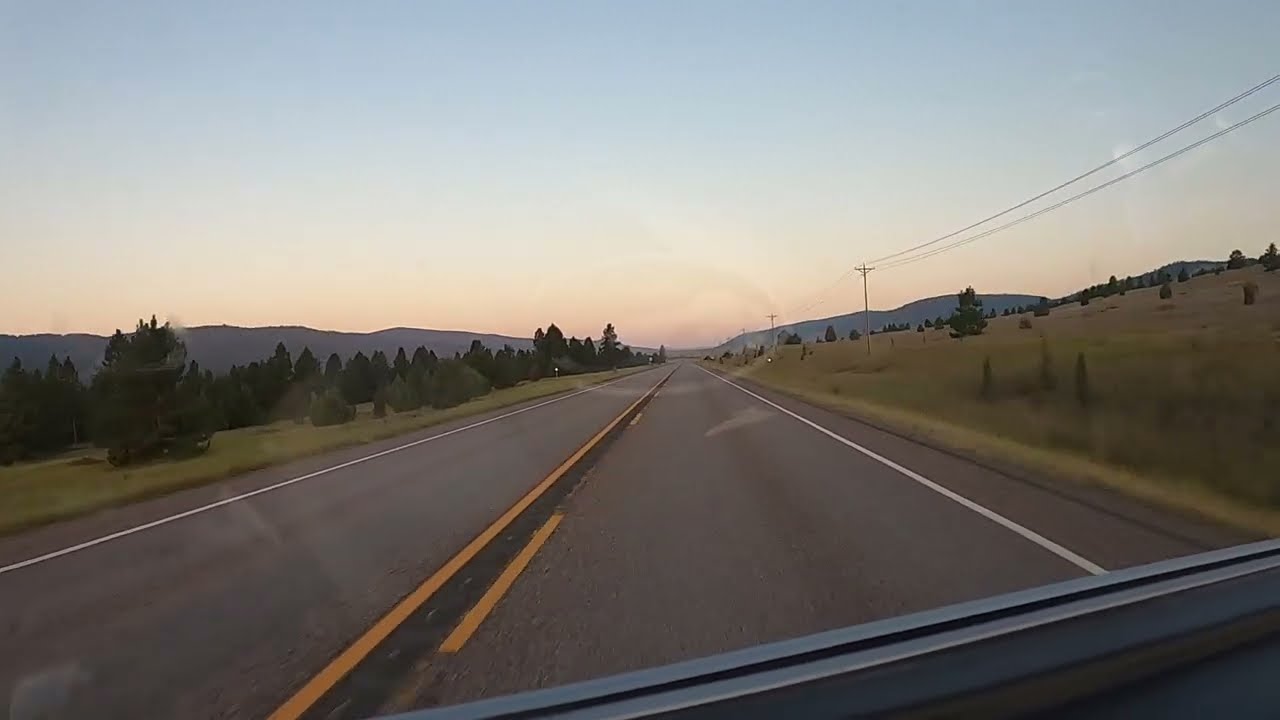The photograph captures the view from inside a vehicle, likely a car or bus, traveling along a two-lane highway. The highway stretches from the bottom of the image up toward the horizon, dividing the scene with a solid yellow line down the middle and a dashed yellow line to its right, flanked by white fog lines on the outer edges. The vehicle is positioned on the right side of the road.

On the right side of the highway, a grassy hill slopes upwards, populated with thin tall grasses and bordered in the distance by a line of telephone poles. These poles appear taller than the surrounding low hills, suggesting that the hills are not particularly high. To the left of the highway, the terrain slopes downwards, leading to a trough filled with closer and larger dark trees. Further left in the background, additional hills or mountains appear as dark silhouettes against the horizon. 

The scene is set under a light blue, hazy sky, with the light condition indicative of either dawn or dusk. The entire vista is viewed through a vehicle windshield, adding a frame of reference to the winding countryside road that recedes into the distance.